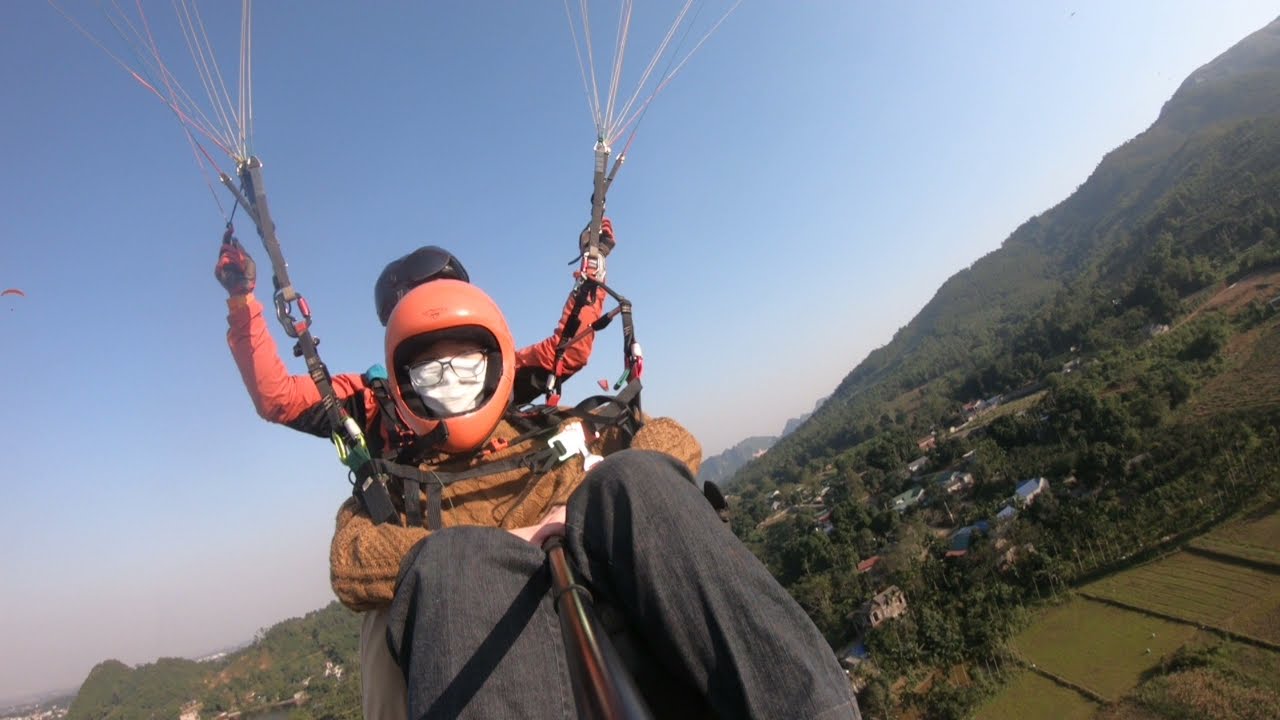The horizontally aligned, rectangular aerial photograph captures two individuals tandem skydiving. The person in the front wears an orange helmet and glasses, along with a brown sweater and black or dark gray jeans. This person's gender is indeterminate. Positioned behind them is another individual with a black helmet, whose face is completely obscured. This person is gripping bars connected to the parachute's suspension lines, indicating control over their descent. They are seemingly in a training scenario, possibly using a life-like dummy, as suggested by the rigid, white plasticine face of the front person. Below, the landscape unfolds into a patchwork of flat green land, dense clusters of trees interspersed with houses, and an elevated mountainous region on the upper right. The backdrop boasts a clear blue sky, free of clouds.